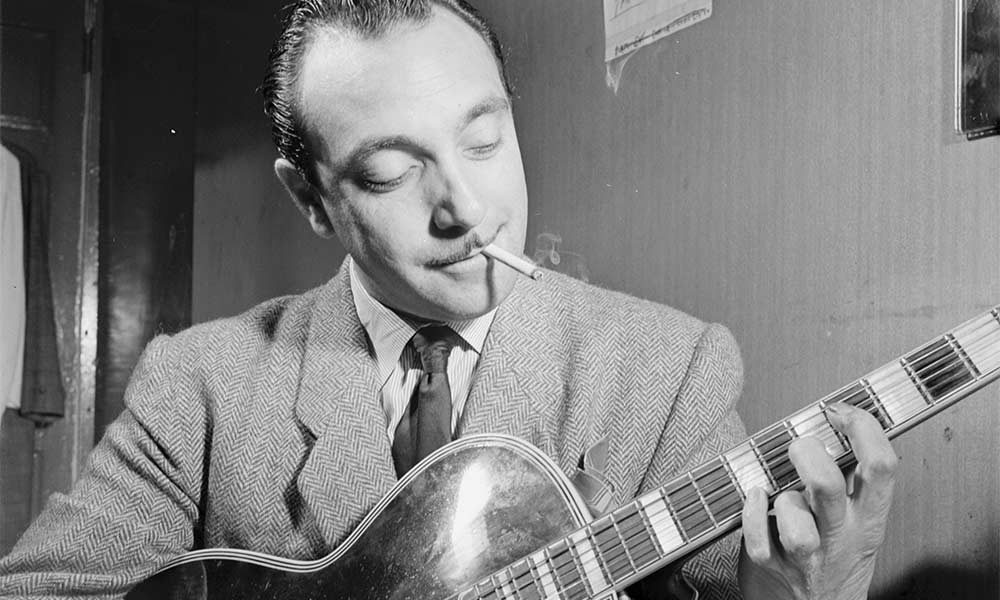This is a close-up black and white photograph of an older man, likely in his late 50s, who is playing the guitar while seated. His hair is slicked back and slightly receding, and he sports a mustache. The man exudes a vintage, retro style and is dressed in a formal three-piece suit with triangular marks creating a textured appearance. He also wears a tie and a collared shirt. He holds a cigarette in his mouth and is smiling with closed lips. One of his wrinkled hands curls like a bird's talons around the neck of his guitar as he plays, indicating his aged experience. The dark-colored guitar features light and dark stripes, though the bottom half of it isn't visible due to the closely framed shot. The lighting highlights his upper body against a dark, nondescript background, adding a dramatic focus on his figure while suggesting a potentially fragile, trailer-like environment. The photograph, devoid of any text, gives a timeless and nostalgic feel, drawing attention to the intricate details of the musician and his setting.